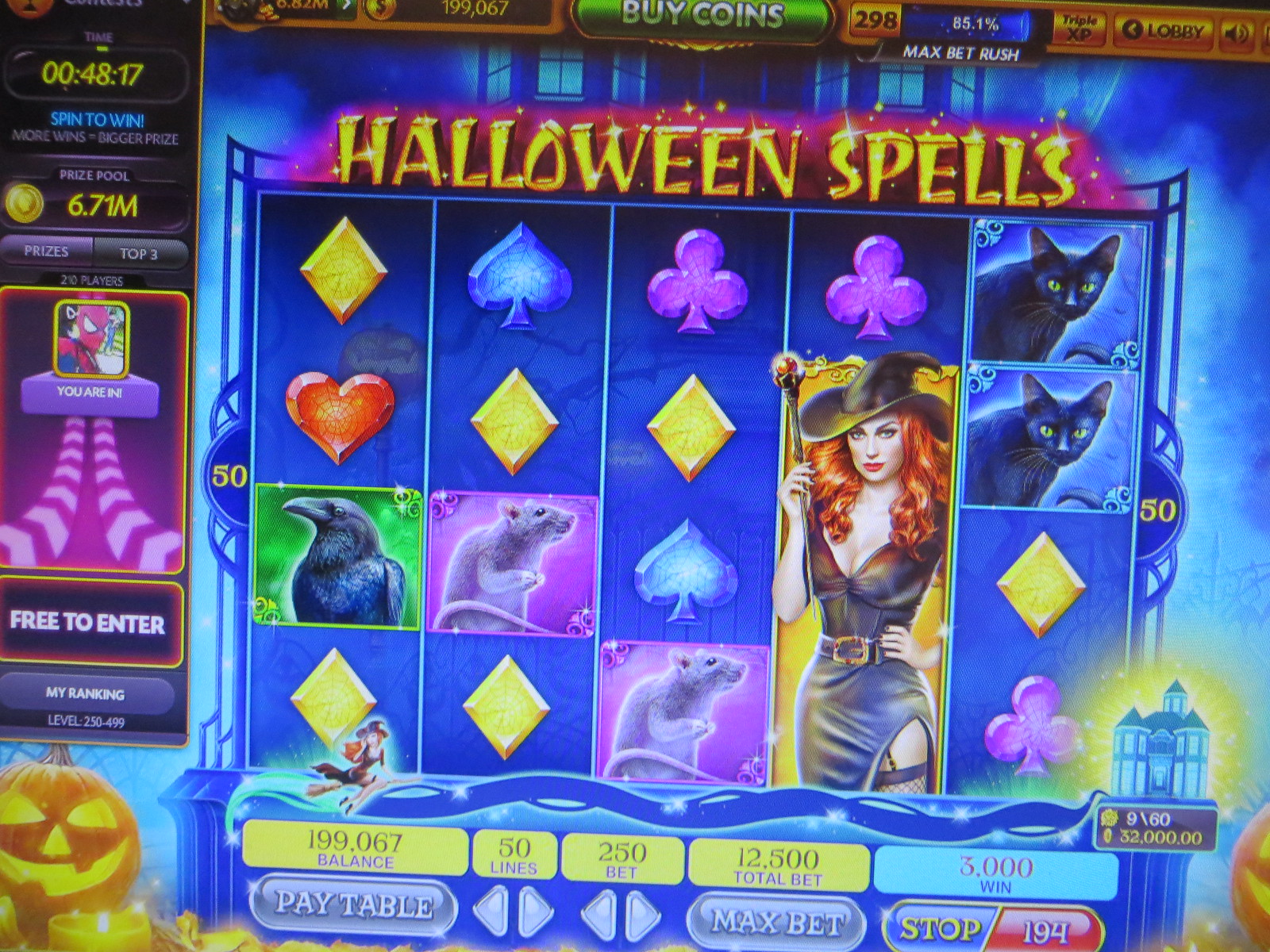The image is a screenshot of a colorful and detailed computer game titled "Halloween Spells," displayed in glittering gold text at the top. Dominating the center of the screen are five columns and four rows populated with various icons such as a yellow diamond, heart, blue spade, crow, rat, and two black cats. Prominently, a red-haired witch dressed in a black hat and gown, holding a red staff, takes up three rows.

At the top center, the screen features a "Buy Coins" option, hinting at the game's gambling nature. The left side displays counters that likely represent scores and balance with values of 195,067 and 199,067. A timer showing "48 minutes 17 seconds" and labels like "Spin to Win" and "Free to Enter" are also visible. The right side includes a "Max Bet Rush" button with an 85.1% indicator above it, alongside other buttons such as "Triple XD," "Lobby," and a speaker icon.

Additional information at the bottom reads "Pay Table," "Max Bet," "Stop," with various other stats such as "250 Bet," "12,500 Total Bet," "3,000 Win," "50 Lines," and rankings that span from level 250 to 499. The bright blue background and colorful icons emphasize the vibrant, engaging style of the game.